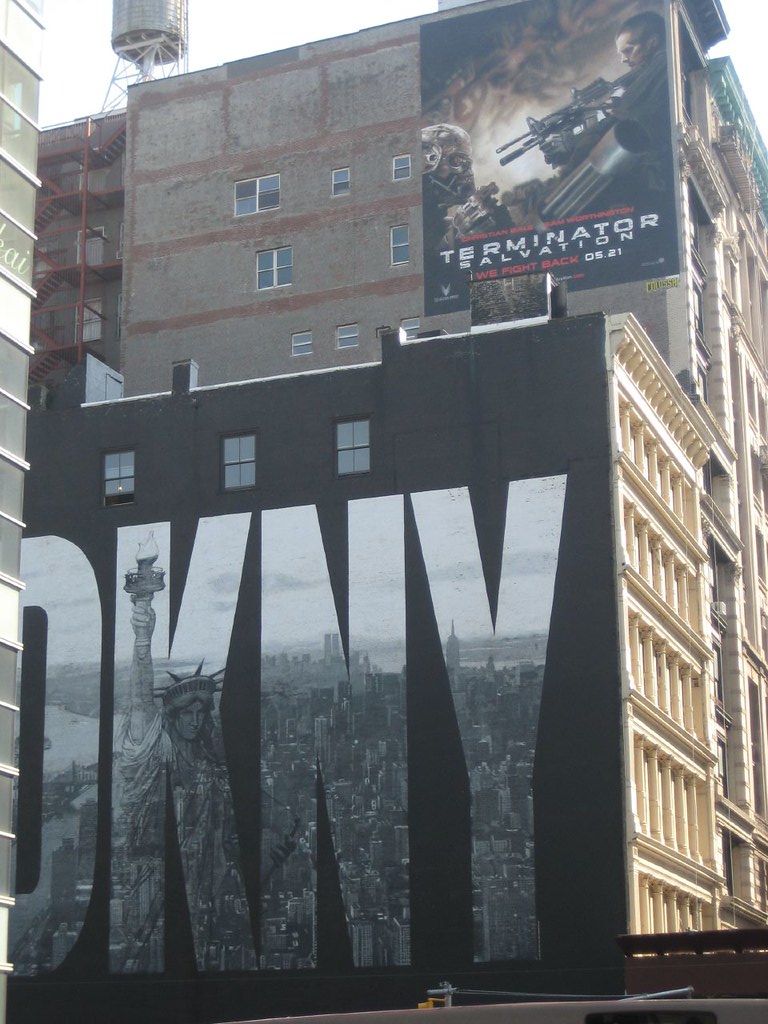This photograph captures the side profiles of two towering buildings in an urban landscape. On the left, a shorter structure is entirely painted black and prominently features the large letters "DKNY" in silver. Inside these letters, an intricate mural depicts the Statue of Liberty alongside a bird's-eye view of New York City, creating a striking visual tribute to the metropolis.

Adjacent to this, a taller, weathered building showcases the aged, worn aesthetic of its exposed brickwork, reflecting a piece of the city's architectural history. On the right side of this building, a massive, eye-catching black poster for the movie "Terminator Salvation" is displayed. The poster features the tagline "We Fight Back" in bold red text, and an opening date of May 31st (531). The graphic depicts a fierce, determined man aiming a rifle at a menacing creature that appears to be a hybrid of human and robot, hinting at the film's intense, action-packed narrative. This juxtaposition of vibrant advertisements and historical architecture encapsulates the dynamic and layered essence of the city.